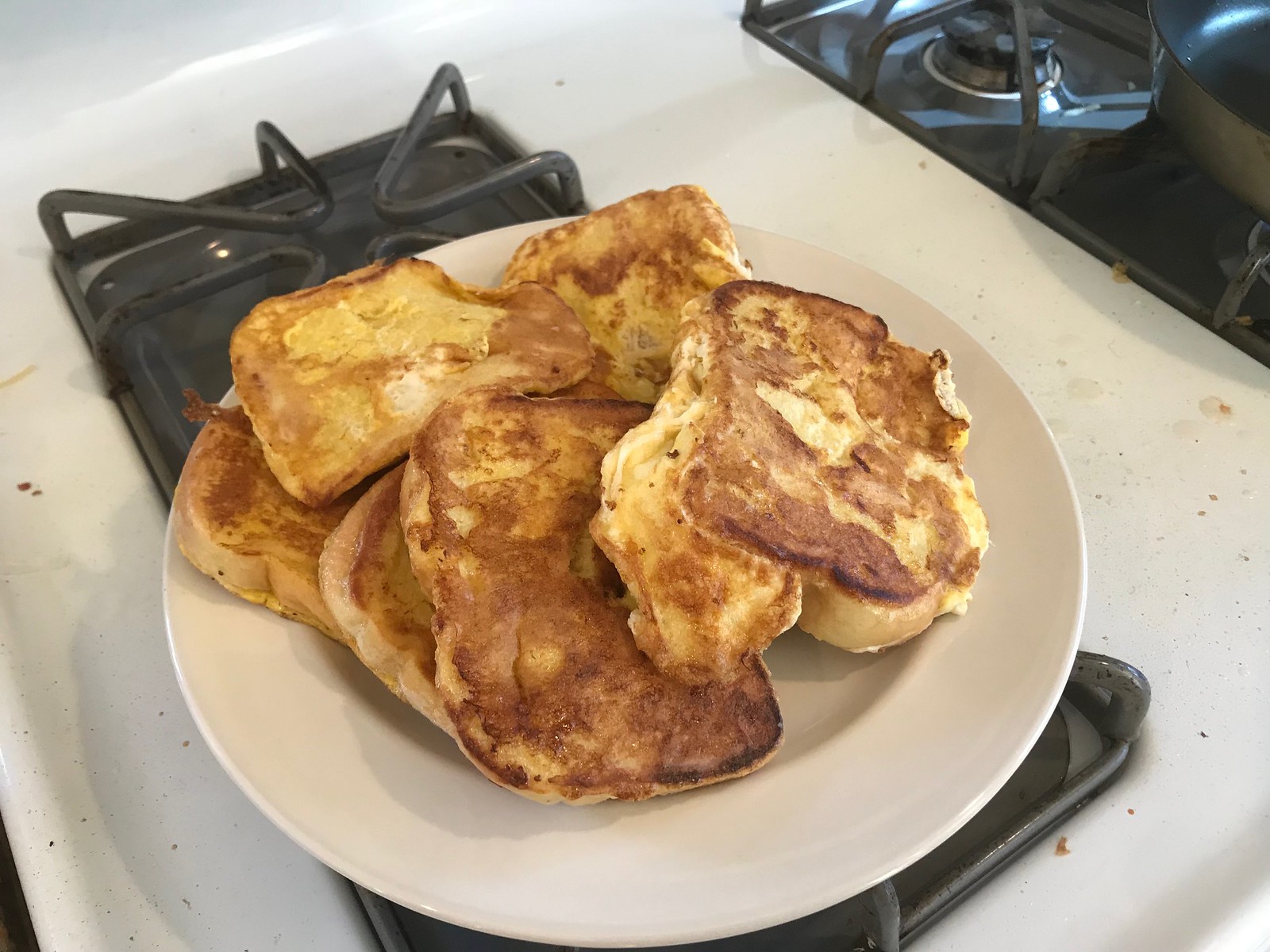The photograph, taken indoors, captures a close-up view of a gas stove with a white surface, which is cluttered with food crumbs and spots. On the upper right, the intricate details of the gas stove burners are visible, showcasing black metal grates and the black and silver center burners. A lidded pan rests on the front right burner. The central focus of this image is a large white plate set on the front burner, holding six fluffy, golden-yellow and brown pieces of what appears to be French toast or very thick, fluffy pancakes. These pieces are not stacked but artfully arranged, casting shadows onto the stove surface. No syrup or additional toppings are present on the French toast. The upper left corner of the photo introduces a white ceramic detail, adding contrast to the overall composition.